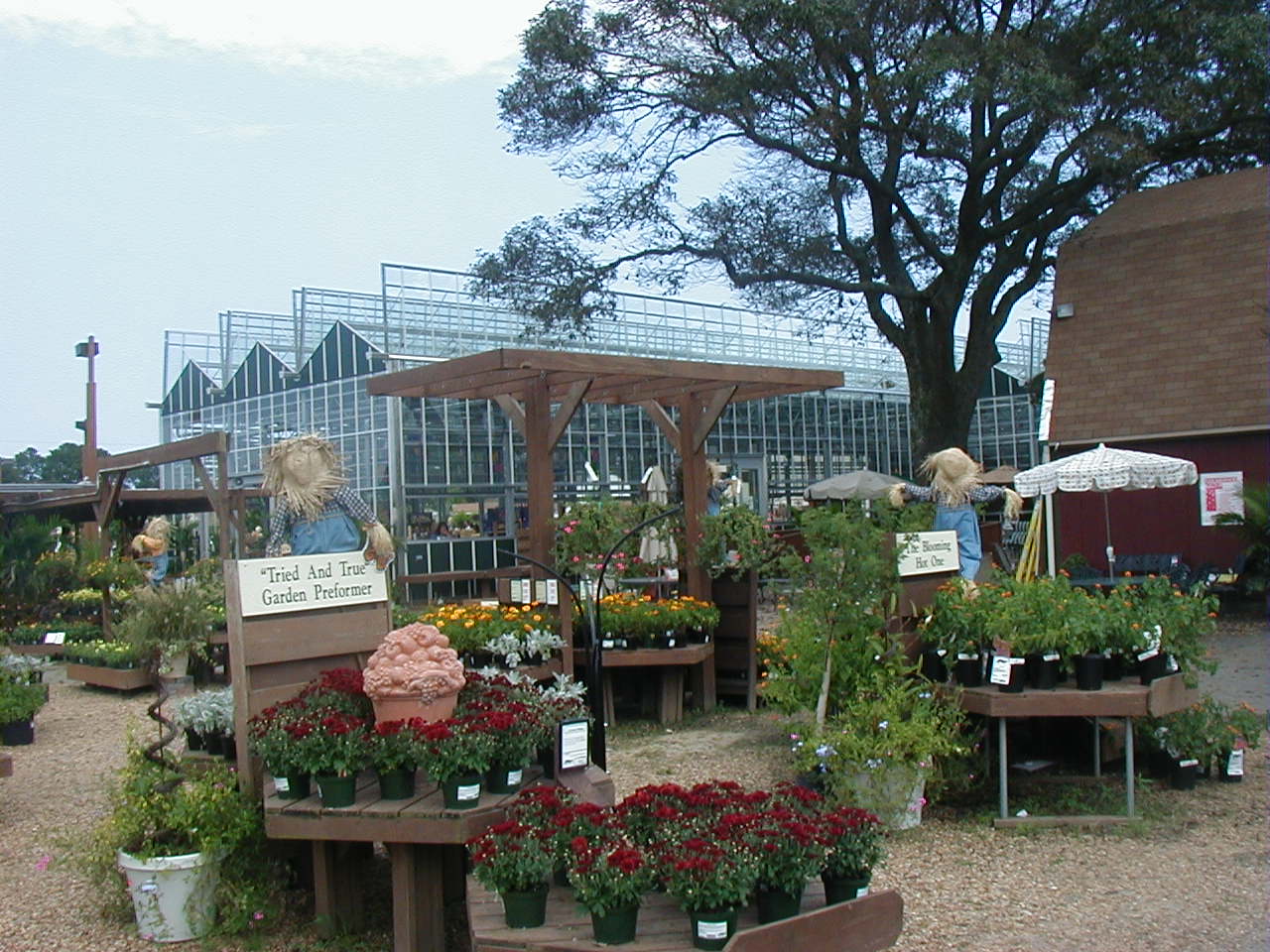This image captures a bustling outdoor plant nursery brimming with vibrant flora under a clear sky. The foreground features a stand of potted mums, some in full red, orange, and yellow bloom, while others are still budding, all accompanied by a sign stating "Tried and true garden performer" — notably with 'performer' misspelled. The nursery grounds are covered in pea gravel, facilitating easy walking among the displays. To the right, a large red building with an expansive roof provides a picturesque backdrop, along with an imposing oak tree casting partial shade. The right side is accentuated with a patio umbrella amidst the plant stands. Scarecrows adorned with informative signs about plant care are scattered throughout. Several trellises support hanging plants, such as Creeping Charlie, and further in the distance, connected greenhouses brim with a multitude of additional plants. Outdoor lights strung overhead add to the inviting ambiance of this vibrant plant haven.